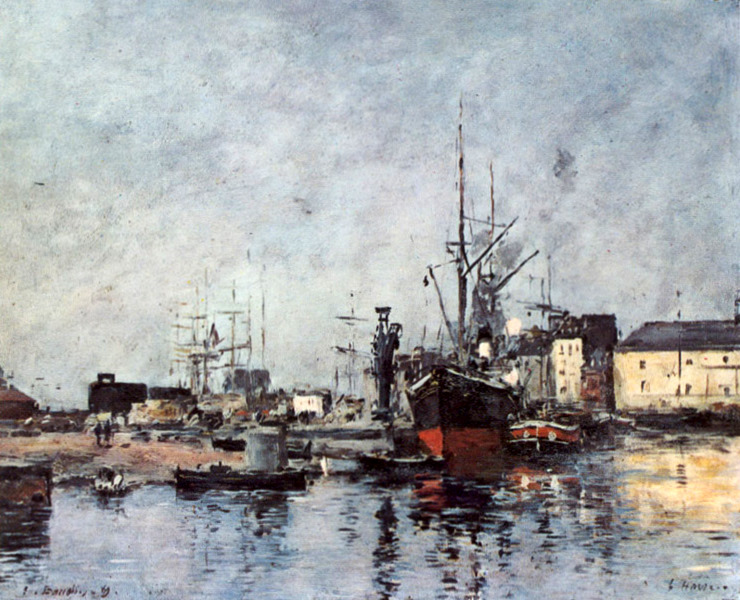This detailed watercolor painting depicts a classic seaport under an overcast sky with gray and white clouds. The reflective water at the bottom of the image captures and mirrors the hues of the surrounding scene, including the reds, tans, and blacks of the ships. Central to the composition is a prominent ship with a red base and a black upper part, featuring masts and rigging but no sails. Beside it, to the right, is a smaller tugboat, also accented in red and black with a white top rim. Farther in the background, a large vessel with white sails adds depth to the harbor view. On the right-hand side stands a large tan-beige building with a black roof, whose reflection also dances on the water's surface. To the far left, two human silhouettes appear to be walking on a dirt mound, contributing to the lively seaport atmosphere. The image, marked by signatures at the bottom left and right (the former partially legible as J-something), captures a vivid, bustling harbor scene replete with intricate details and engaging textures.